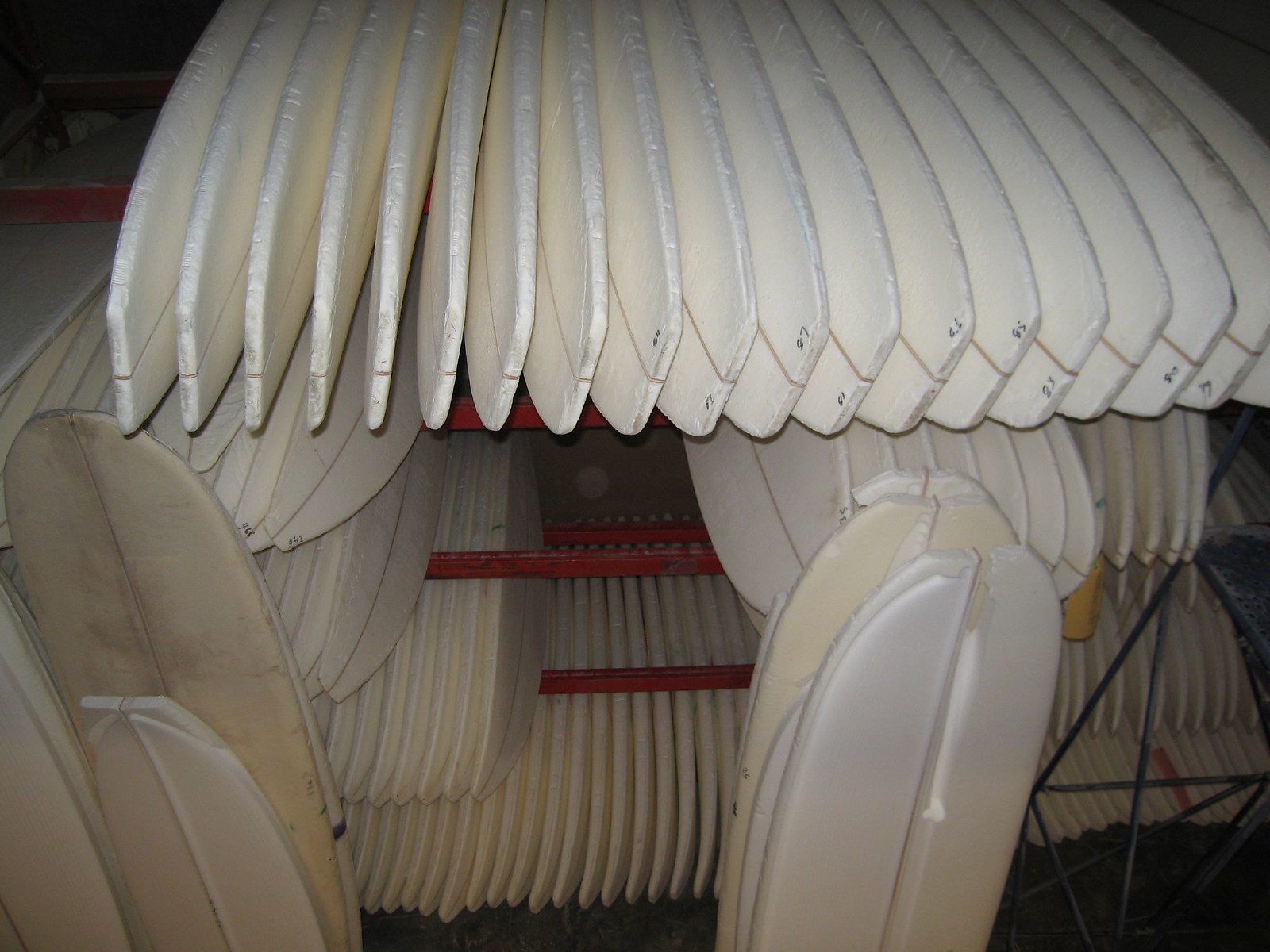This color photograph captures a largely white scene featuring an intricate arrangement of what appear to be unpainted and unfinished boogie boards or styrofoam surfboards. The boards are meticulously organized on red metal racks, creating a striking visual pattern. At the top of the image, the boards fan out vertically, resembling the petals of a flower or the spokes of a merry-go-round. Below this primary layer, additional layers of boards are visible, also fanned out but separated by gaps defined by the structure of the red metal racks. Some boards lean forward from the racks, either in the middle right portion of the image or towards the left, adding a touch of asymmetry to the otherwise structured composition. In the lower right corner, a black metal triangular frame can be seen, adding contrast to the predominantly white and red scene. There are no people, animals, buildings, or motorized vehicles in this image, further drawing attention to the stark and repetitive forms of the boogie boards.